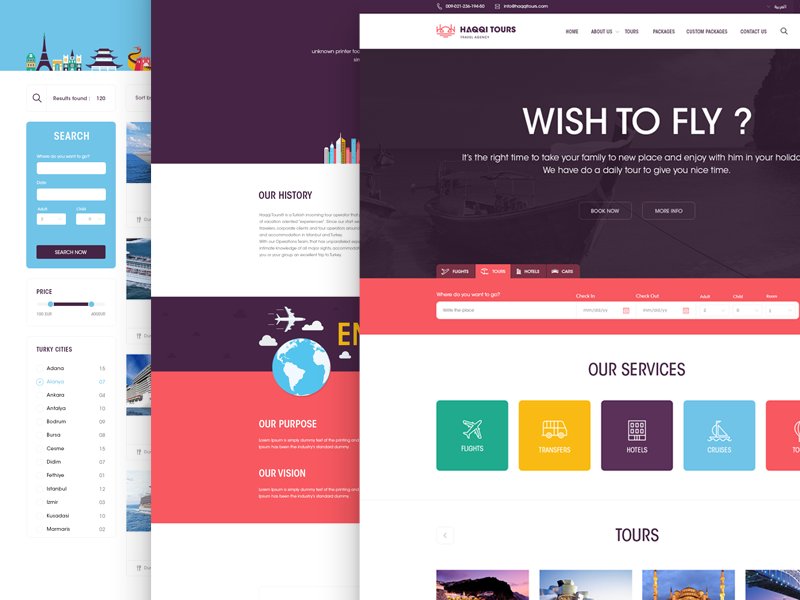This image is a screenshot from the Haqqi Tours website, showcasing three layered web pages. The topmost page appears on the right side, angled slightly to the right as if emerging from the center. In the top-left corner of this page, the site’s name "Haqqi Tours" is displayed prominently in large letters, accompanied by a red temple symbol logo. This page is titled "Our Services and Tours," and features a prominent banner at the top with the phrase "Wish to Fly." Below this banner, a section labeled "Our Services" includes small icons representing various travel options such as flights, hotels, and cruises, with a subsection specifically for tours.

Beneath the top page, another page titled "Our History" is partially visible, hinting at detailed information about the company’s background and legacy. The third page, positioned at the very back and partially obscured, only reveals a search box on the left side that prominently displays prices, suggesting functionality for users to search and compare travel costs. The layered arrangement of the pages provides a dynamic, in-depth look at the different sections of the Haqqi Tours website, emphasizing the company’s comprehensive travel services.